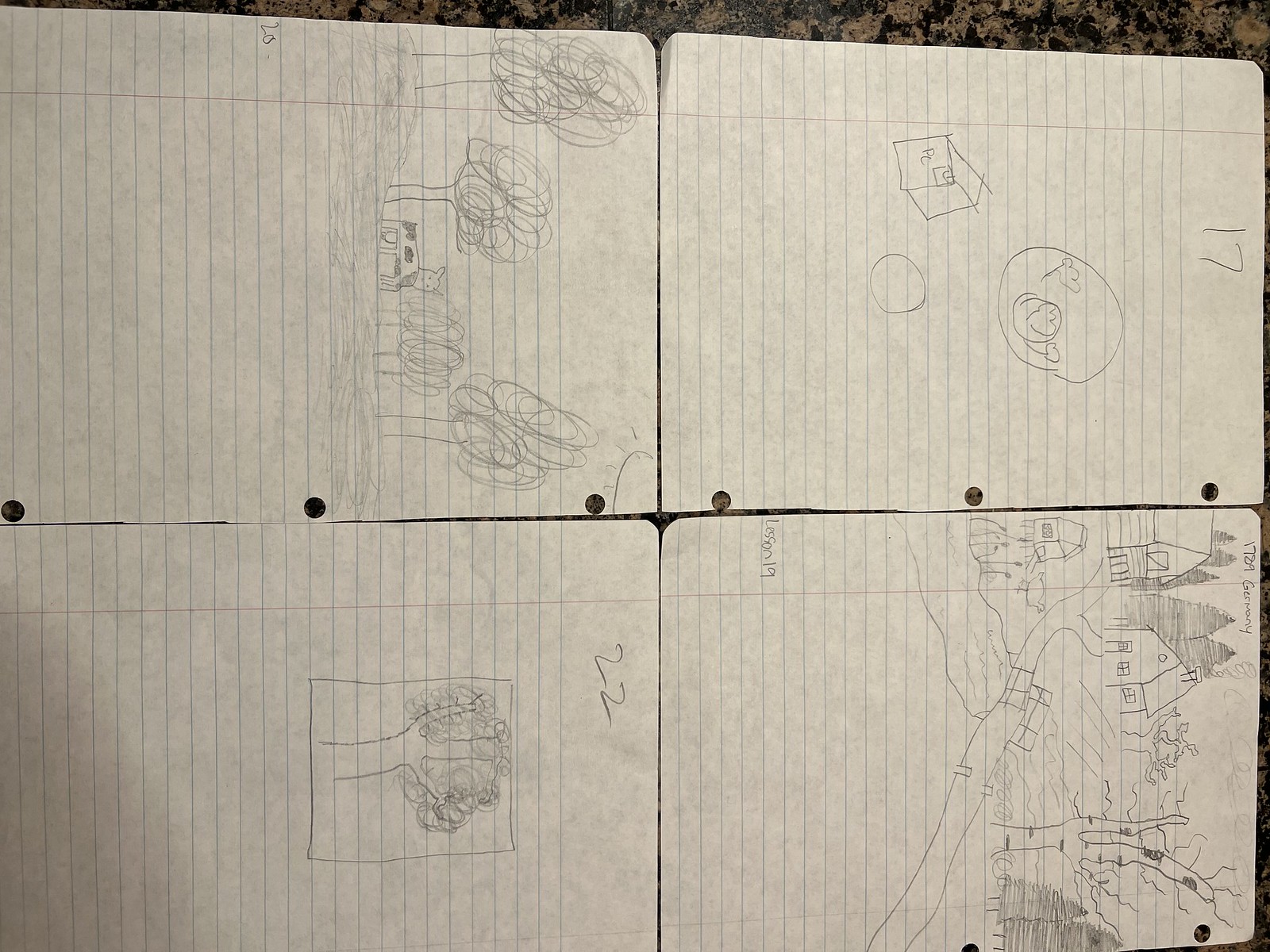This photograph showcases four meticulously drawn pencil sketches on standard lined 8 1⁄2 by 11-inch paper, displayed against a textured countertop. 

- The upper left sketch features a detailed depiction of a plate of food contained within a box, capturing intricate details and textures. 
- The upper right sketch presents a picturesque scene with a house approached by a winding path that crosses a bridge over a serene river. The composition includes multiple houses and lush trees set against an expansive natural backdrop.
- The bottom right sketch portrays a sturdy tree, possibly an orange tree, showcasing the artist's attention to its intricate branching and foliage.
- The bottom left sketch illustrates a pastoral landscape with a few trees and a lone cow standing on a grassy hill, rendered in shades of black and white.

Each drawing demonstrates a commitment to detail and careful shading, reflecting the artist's skill and dedication to creating lifelike representations using only pencil.